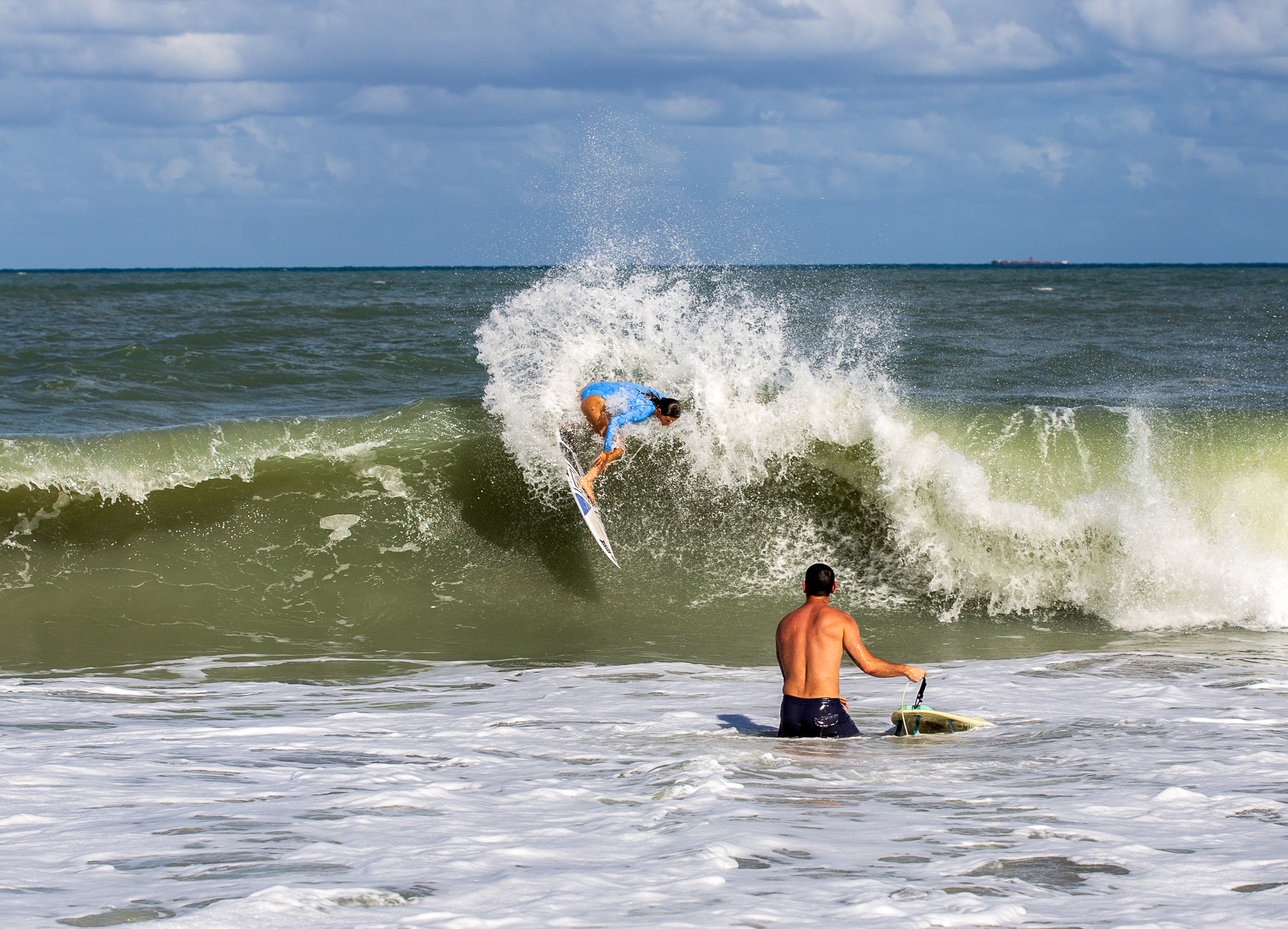The photograph captures a dynamic ocean scene with two surfers in focus. In the foreground, a shirtless male surfer stands, wearing dark blue swim trunks and holding a white surfboard. He appears to be watching a female surfer who is riding the crest of a striking olive green wave. The female surfer, wearing a light blue bodysuit, has dark brown hair and is balanced gracefully on her white surfboard adorned with dark blue shapes. The water around them is rough, with white caps and foam, enhancing the sense of action and movement. Off in the far background, the ocean extends, dark blue-green in color, with the sky above scattered with clouds. There is a suggestion of some distant structure, possibly buildings or a shipping vessel, subtly visible on the right-hand side against the horizon.